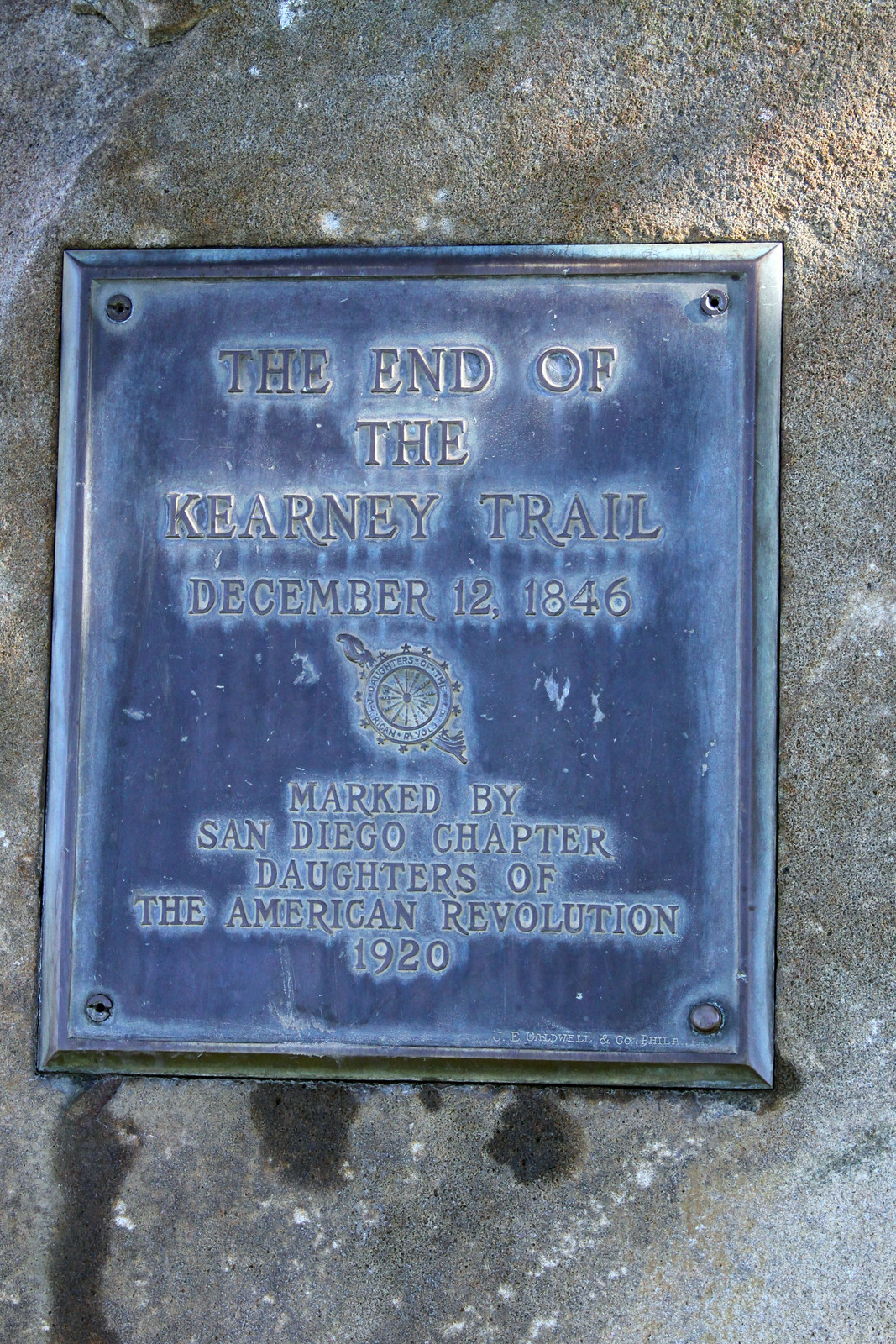This outdoor photograph, taken in portrait orientation, captures a weathered metal plaque affixed to a rough stone wall with patches of moss. The plaque, framed by slight carvings and secured with bolts at each corner, bears oxidized and discolored features that reflect its age. The inscription prominently displays in raised, dark gray letters with white weathered outlines: "The End of the Kearney Trail, December 12, 1846." Below the inscription, a circular seal resembling a compass, encircled by stars and the phrase "Daughters of the American Revolution," is engraved. Underneath the seal, the text reads, "Marked by San Diego Chapter, Daughters of the American Revolution, 1920." In the lower right corner, it further notes the plaque's creator, "J.E. Caldwell and Co., Philadelphia." Despite its weather-beaten and faded condition, the detailed engravings document a significant historical marker, resonating with the legacy of the past.